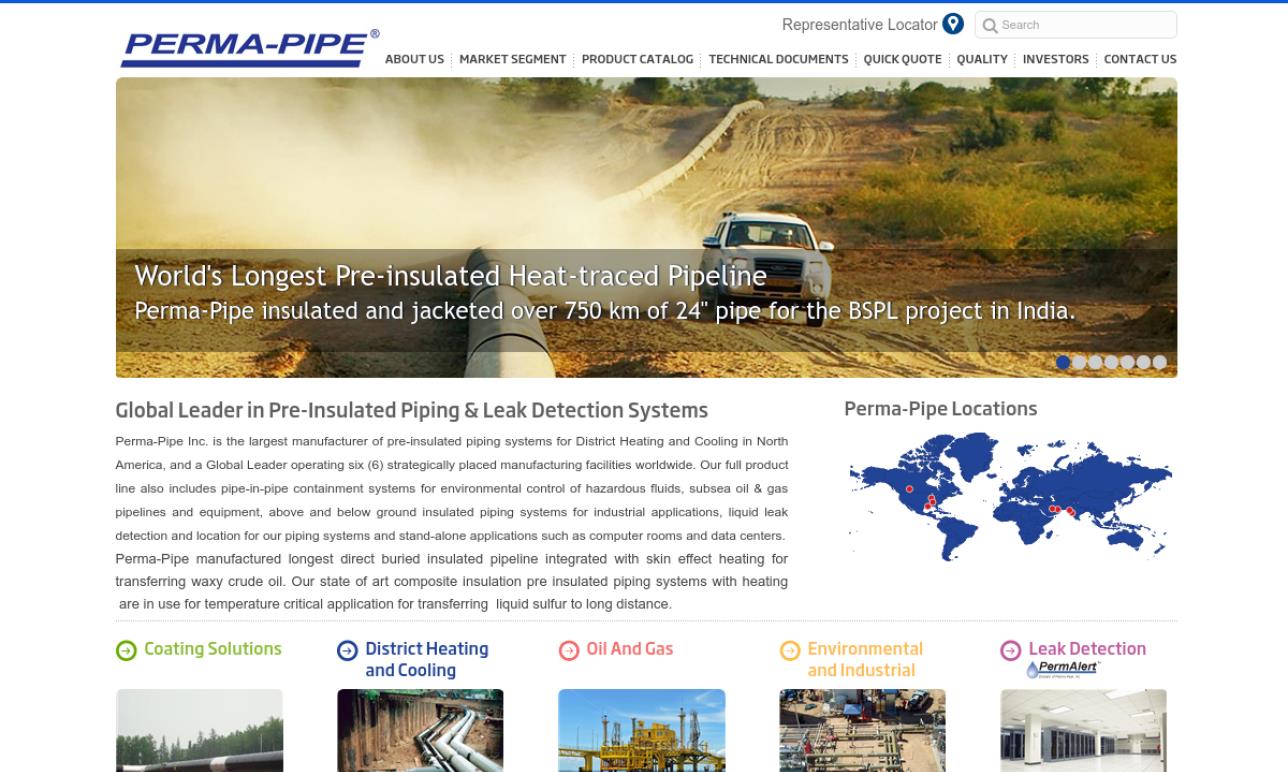The image prominently features the Permapipe logo in the top left corner. The categories displayed include "About Us," "Market Segments," "Product Catalog," "Technical Documents," "Quick Quotes," "Quality," "Investors," and "Contact Us." Additionally, the image highlights the world's longest pre-insulated and heat-traced pipeline, a notable project where Permapipe insulated and jacketed over 750 kilometers of 24-inch pipe for the BSPL project in India. As a global leader in pre-insulated piping and leak detection systems, Permapipe Inc. is recognized as the largest manufacturer of pre-insulated piping systems for district heating and cooling in North America. The company operates six strategically located manufacturing facilities worldwide. Permapipe's product line includes pipe-in-pipe containment systems for the control of hazardous fluids, as well as subsea oil and gas pipelines and equipment.